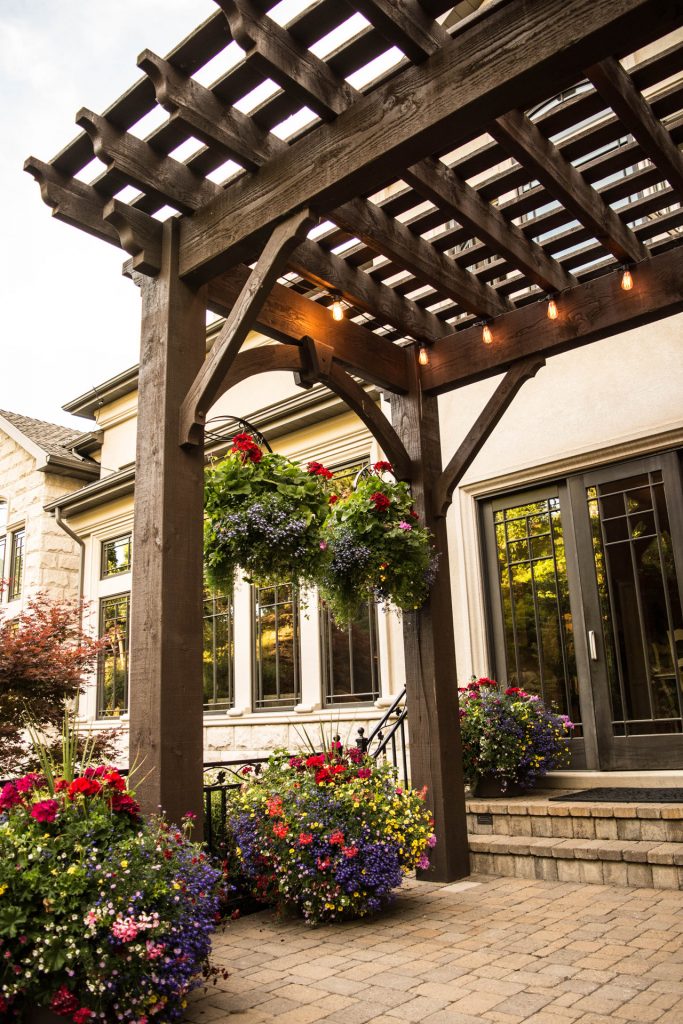This image depicts a luxurious entryway, possibly of a house, from the perspective of someone standing a few feet back, right in front of the steps leading to the main door. The elegant entry features a two-step staircase made of gray bricks that ascends to a set of double doors with brown frames and long rectangular windows. The building itself appears to be constructed from beige cream-colored brick stone, with vertical windows aligning the left side of the entrance.

Dominating the foreground is a large wooden archway, a pergola-like structure with brown beams and a lattice pattern on top. The overhang features horizontally and vertically arranged wood slats, allowing dappled sunlight to filter through. Hanging from the left side of the archway are metal arches adorned with potted plants bursting with red, pink, purple, and white flowers. Similar flower arrangements are positioned below the hanging baskets and along the black metal railing that flanks the steps.

Adding to the charm, warm amber-colored lights dangle from the pergola, complementing the tranquil ambiance of the overcast sky above. The scene is set against the backdrop of what seems to be a sandy-colored stone patio area, enhancing the sophisticated and welcoming atmosphere of the entrance.